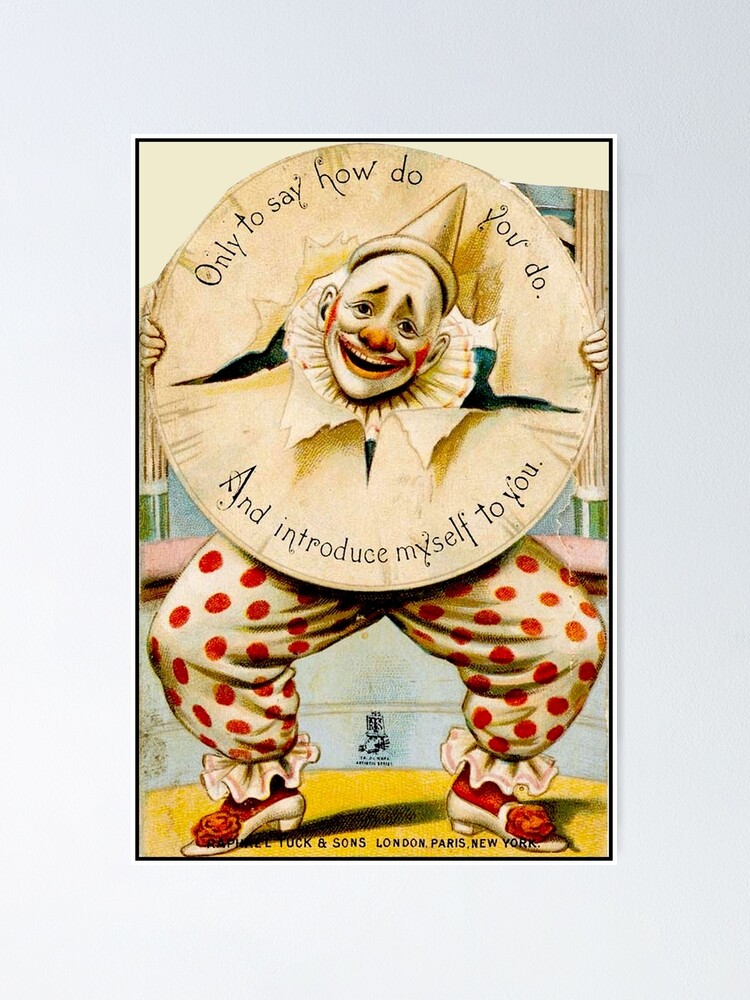This image is a detailed, contemporary drawing reminiscent of an old circus advertisement or an antique greeting card. It features a clown with a distinct, silly appearance, likely positioned on a stage or platform. The clown's head bursts through a cream-colored paper-covered hoop, which has text on it: "Only to say, how do you do?" at the top and "and introduce myself to you," at the bottom. The clown sports a red nose, red cheeks, and a red-painted smile against a white face, with a bald head topped by a cone hat. He wears a green shirt with a white ruffle collar, baggy beige pants decorated with red polka dots and ruffles at the ankles, red socks, and white shoes with red flowers on the tops. Below the clown's feet, the text reads, "Tuck & Sons, London, Paris, New York." The entire image is bordered by a gray background, enhancing its vintage aesthetic.